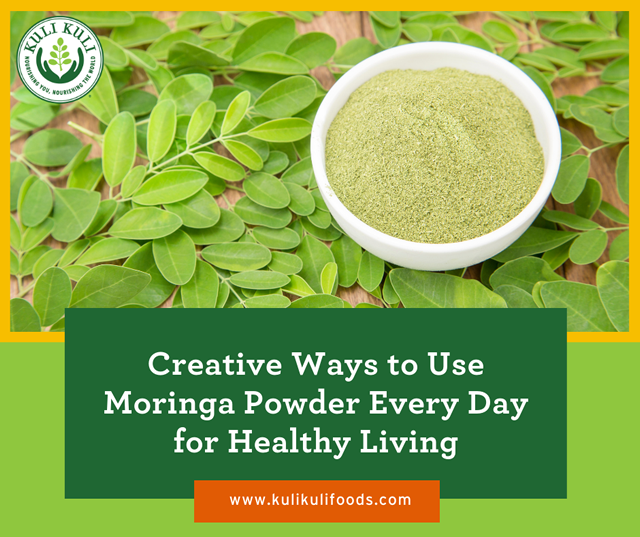The advertisement features a vibrant green and yellow color scheme, centered around the benefits of moringa powder. At the top of the image, there's a professional photograph outlined in yellow, showcasing a white bowl filled with green moringa powder. This bowl is artistically situated on a surface adorned with a spread of green leaves, adding a decorative touch indicative of moringa leaves.

In the top left corner, the Kuli Kuli Foods logo is displayed prominently, depicting two hands cradling a branch symbolically. Below the logo, the text "Creative ways to use Moringa powder every day for healthy living" is clearly written on a green background with white lettering. Toward the bottom right, there is an orange box with white text that directs viewers to visit www.kulikulifoods.com.

The image ties together various elements harmoniously; the bowl's placement on the leaves, the highlighted moringa powder, and the Kuli Kuli branding elements, creating an engaging visual narrative that promotes the everyday use and health benefits of moringa powder.